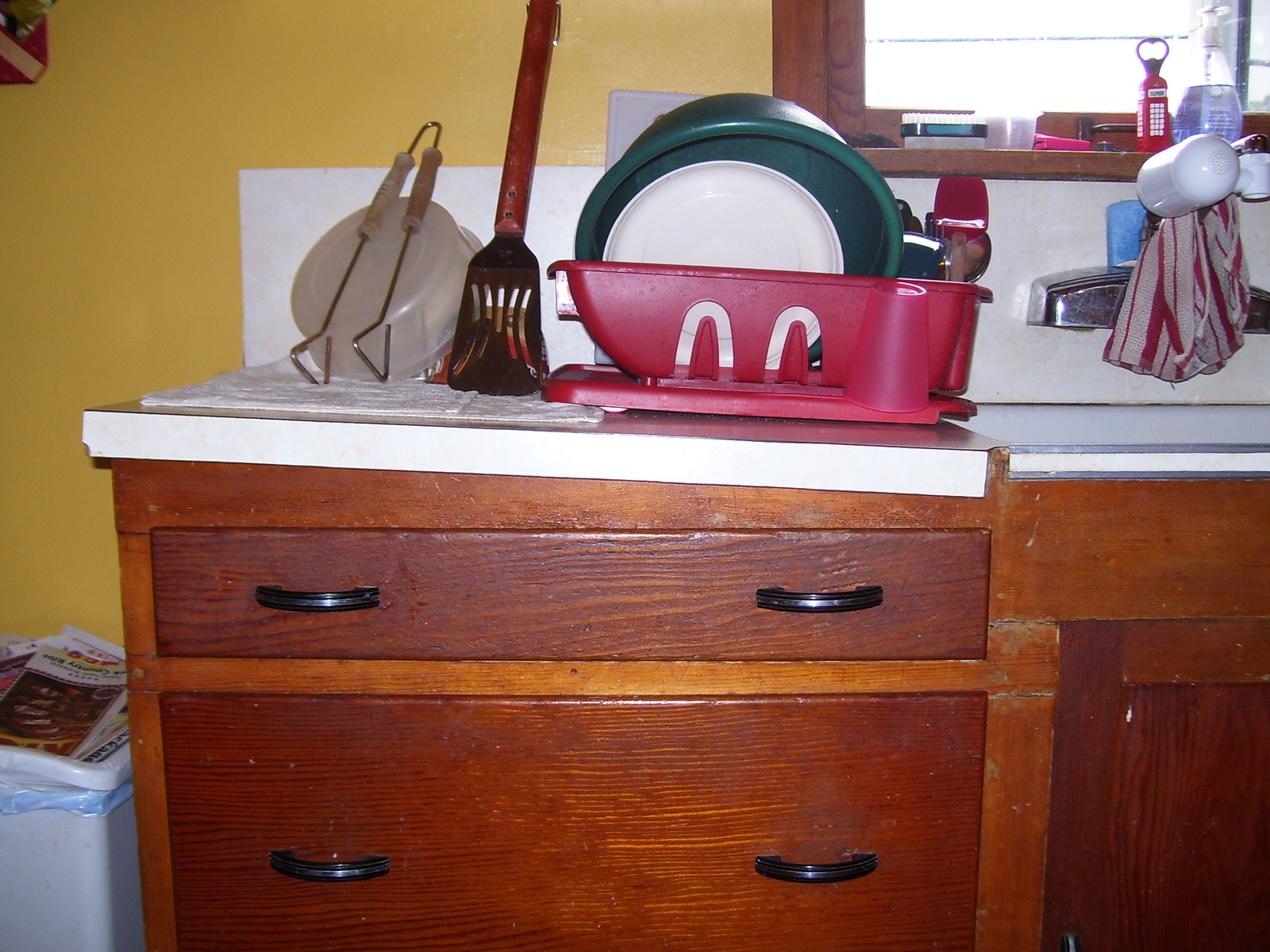The photo captures a cluttered kitchen scene, taken indoors. A dull yellow wall serves as the backdrop, featuring a wooden window pane situated in the upper right corner. The window's sill holds several items, including beauty products like cologne, a little plastic cup, and other indistinguishable objects. Beneath the window is a white rectangular structure fitted with a stainless steel sink faucet, around which a gray and red rag is tied.

The edge of the sink is occupied by a red dish drainer filled with an assortment of dishes, including a white plate and a dark green bowl. On the counter beside the dish drainer lies a spatula, a pair of tongs, and a plastic bowl placed on a white towel. Below this countertop, a wooden cabinet with multiple drawers features two black handles on each drawer. Adjacent to the cabinet on the left, a white trash can overflowing with paper and newspapers can be seen, adding to the kitchen's lived-in atmosphere.